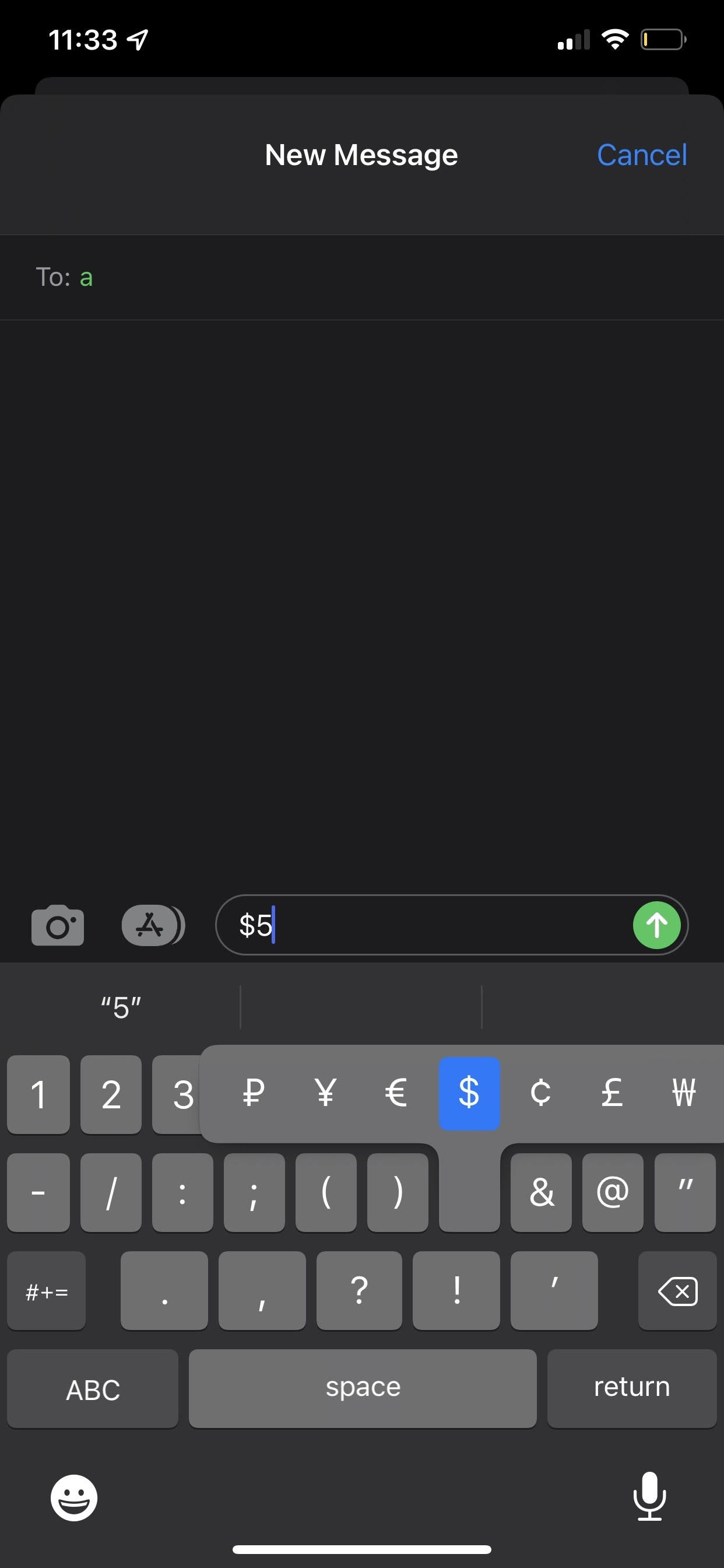The image displays a messaging app interface at 11:33, with two signal bars on the right and a full Wi-Fi signal. The battery indicator is critically low, almost empty with just one or two pixels left. A popover area at the top says "New Message" with a cancel button to its right. The recipient field shows "To: A" in blue text, followed by a large blank space beneath it. Below the blank space, there are icons for the camera, the Apple App Store, and an input field. The input field contains "$5" with the cursor positioned after the number. Adjacent to the input field is an up arrow for sending the message.

Below this input field, the dollar sign "$5" is quoted again. The keyboard is open and displays various currency symbols, the dollar sign is highlighted in blue, indicating it is about to be selected. The rest of the keyboard appears standard, with a variety of options for currency symbols. At the bottom of the screen, there is an emoji icon on the left and a speaker icon on the right. The app's interface features a palette of blacks and grays, with lighter gray for the keyboard keys and white for the text.